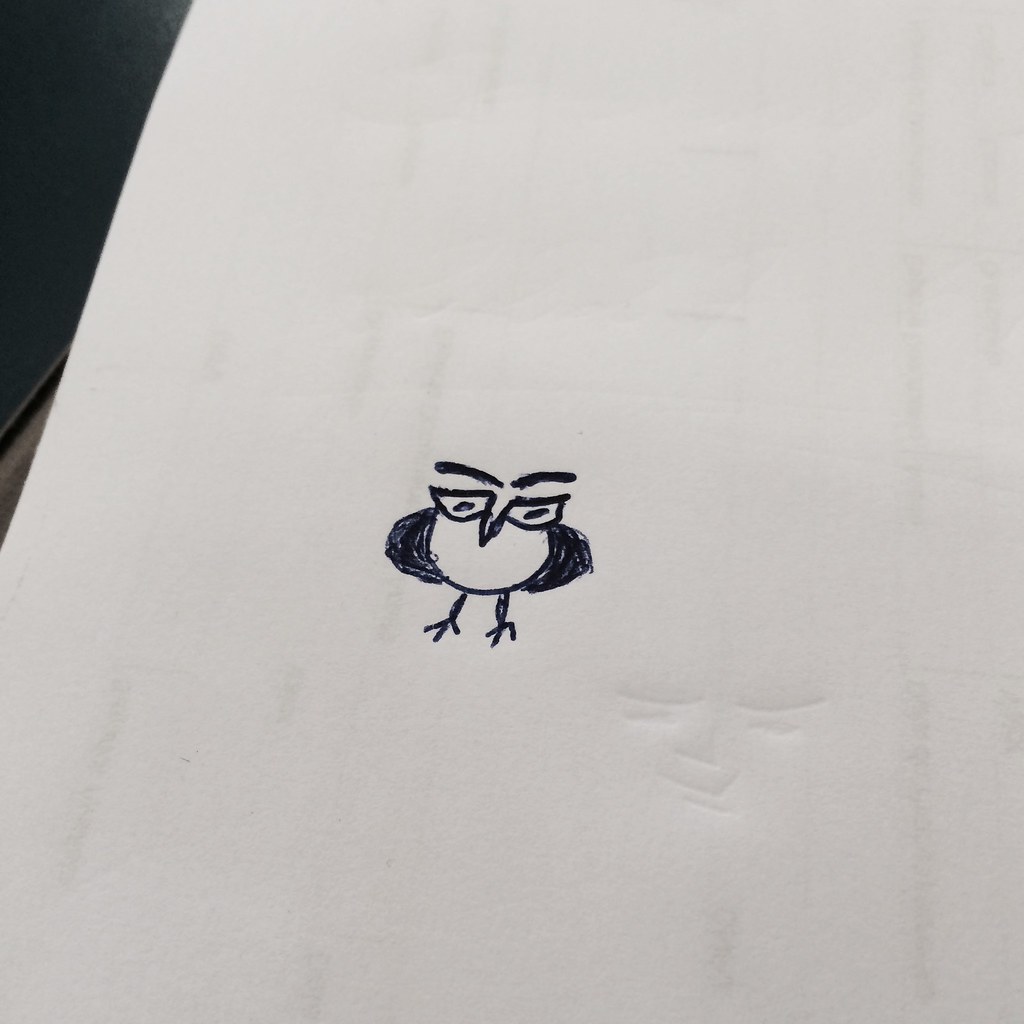This is a photograph of a hand-drawn sketch of an owl on an off-white piece of paper, occupying approximately 90% of the frame. The paper shows indentations of a face drawn on another sheet placed above it. The sketch, created possibly with an ink pen or marker, features a round-bodied owl. It has two distinct eyes, each positioned on either side of a V-shaped nose. Unattached, furry eyebrows appear above the eyes. The owl's wings are moon-shaped and shaded in black. From the bottom of its body, two legs extend, each with three distinct toes. In the top left corner of the frame, the paper rests on a dark surface, partially visible underneath.